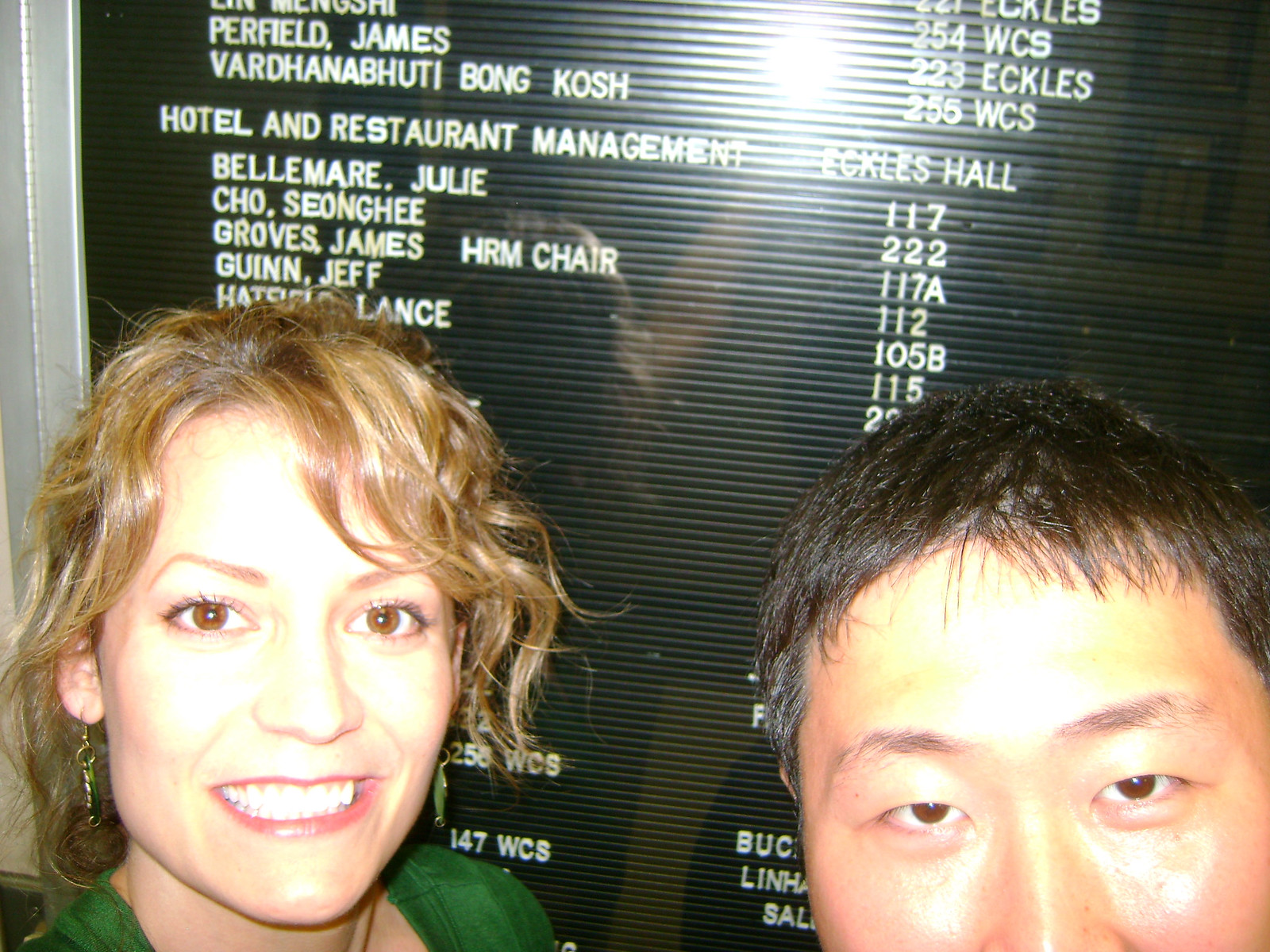This color photograph, in landscape orientation, features a selfie-like close-up of a smiling woman and an Asian man against a black magnetic board adorned with white text. The image is shot from a slightly downward angle, capturing the woman in the bottom left corner; she has short, blonde curly hair, brown eyes, and is dressed in a green top with green earrings. In the bottom right corner is the man, whose face is slightly cropped out of the frame; he has short black hair and brown eyes. Both individuals are looking directly into the camera. The blackboard behind them displays various names and office numbers, including those associated with hotel and restaurant management, such as "Perfield James," "Fardhana," and "Groves, James, HRM Chair." The setting appears to be inside an office building, and the image emits a photographic realism style, often typical of candid, event-related portraits. The overall color palette includes shades of gray, black, white, brown, pink, and green.